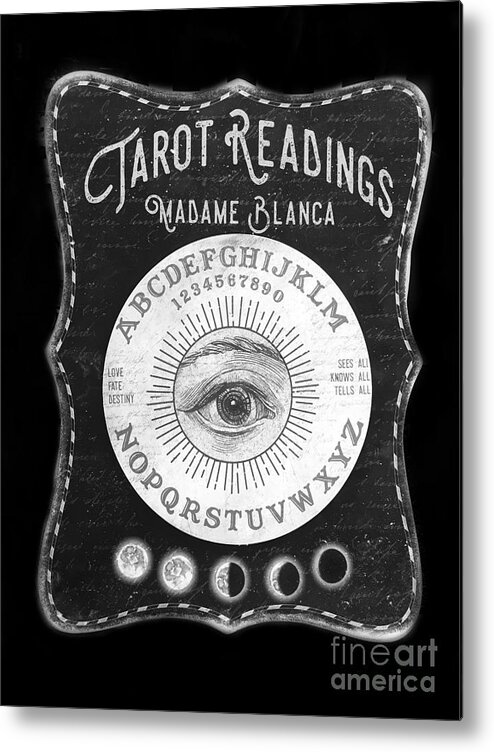The image is a detailed black and white poster featuring an intricately designed advertisement for tarot readings by Madame Lock. Central to the design is a white circle with the alphabet arrayed around its circumference, segmented into A-M at the top and N-Z at the bottom, and numbers 1 through 9, and 0 beneath the alphabet. In the very center of this circle is a prominent human eye, encircled by rays emanating outward, symbolizing a sun-like visage. The top of the poster boldly displays "Tarot Readings" followed by "Madame Lock" in elegant white lettering. Flanking the central circle, on the left it reads "Love, Fate" and on the right "Sees All, Knows All, Tells All," highlighting the mystical nature of the services offered. At the bottom, there are five moon phases transitioning from full moon to a completely blacked-out moon, representing the lunar cycle. The bottom right corner is marked with "Fine Art America" in light gray, indicating the artist or publisher. The overall design suggests an old-timey, mystique-filled advertisement, rich in symbolic imagery and text.